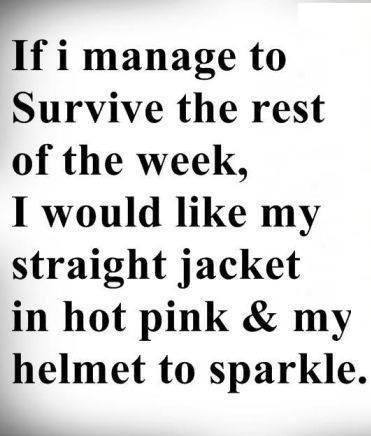The image, likely sourced from a meme or social media post, features black text on a predominantly white background, which has faint shadowing in the corners adding a subtle gradient towards black. The text reads, "if I manage to survive the rest of the week I would like my straitjacket in hot pink and my helmet to sparkle." The formatting has a few peculiarities: the first "I" is lowercase despite following "if," making it a grammatical error in an otherwise run-on sentence. The font used is Times New Roman, and the letters exhibit noticeable JPEG artifacting, particularly around their edges. Additionally, there's an unexplained white box in the top right corner of the image. This whimsical and somewhat humorous text seems to convey a desire for a touch of femininity and sparkle in an otherwise dire or stressful scenario.